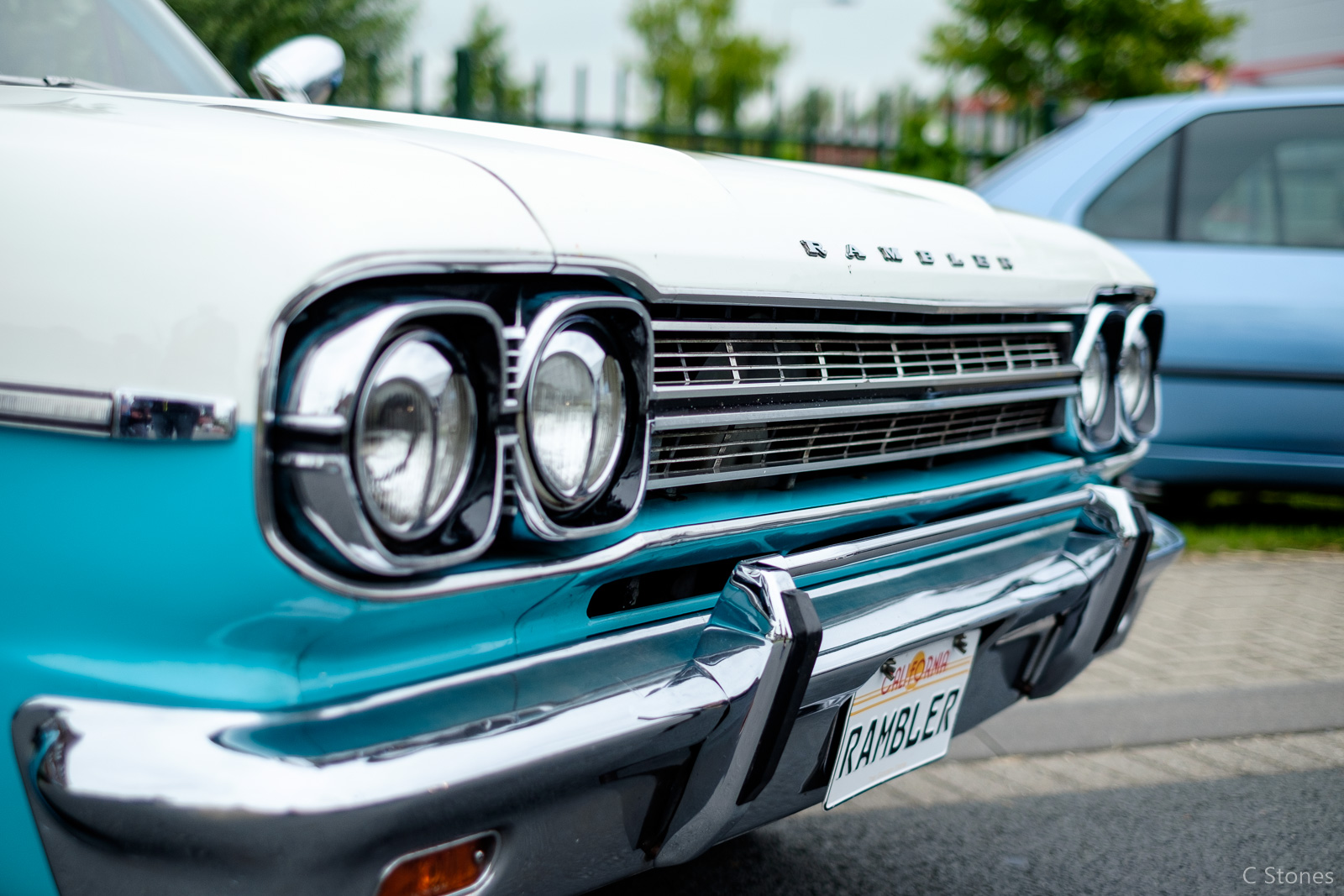This photograph captures the front end of an older Rambler car parked on pavement or brick. The vehicle features a striking design with a white hood and a light sky-blue section wrapping around the fenders. The chrome elements, including a silver bumper, four headlights, and a silver grille, add to its vintage appeal. Prominently displayed in the center of the bumper is a California license plate with the word "Rambler" embossed in red letters. The front also bears the name "Rambler" on the hood. A side view mirror is visible on the upper left part of the image, and yellow warning lights are present on the bumper. In the background, there is another blue car, likely an ordinary model. Beyond the cars stands a black iron fence, and further in the blurred distance, several trees are visible under a grey sky. The lower right corner of the image is marked with the name "C. Stones." The overall scene is devoid of people, and it appears to be a cloudy day with no direct sunlight.